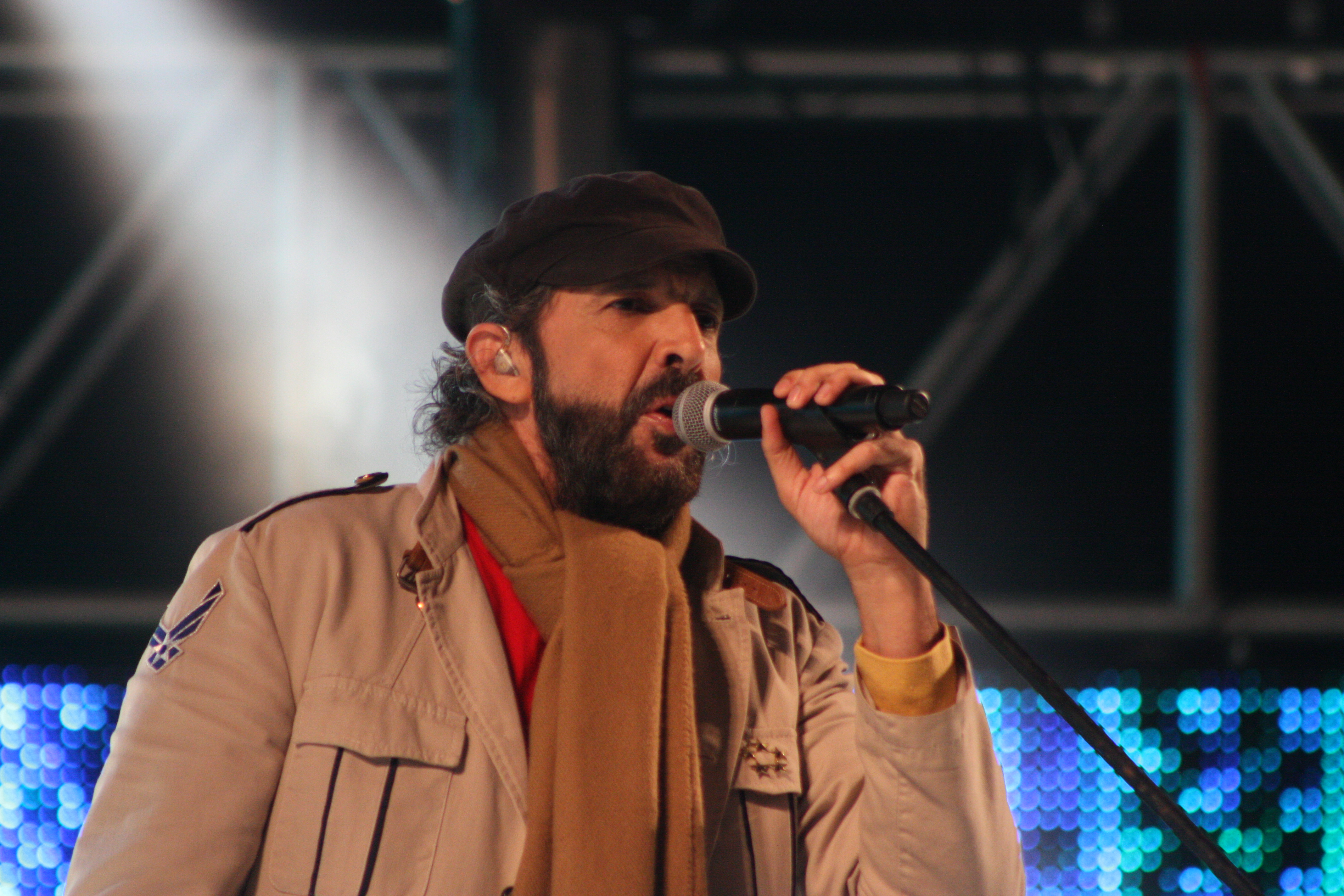The image captures a man in the 45-50 age range, passionately singing on stage. He's holding a microphone close to his lips with his left hand, and the mic is also attached to a stand. He's donned in a distinctive black newsboy cap that sits firmly atop his head, with an earpiece visible in his right ear. His rugged appearance is accentuated by a thick beard and a brown scarf wrapped around his neck. Completing his ensemble is a tan, military-style jacket adorned with various patches, including what looks like an Air Force logo on the right side. The background features the structural elements of the stage, illuminated by blue lights at the bottom, enhancing the overall atmosphere of the performance.